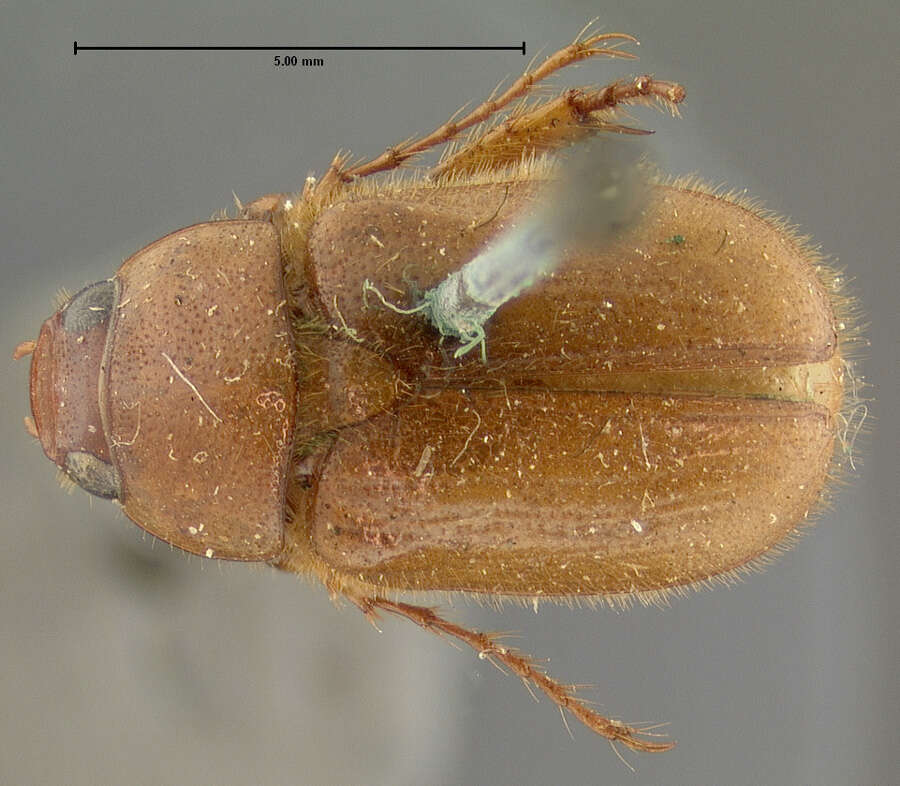This detailed close-up photograph, likely taken through a microscope, features a medium brown beetle as its central subject, positioned horizontally and dominating the image. The beetle, facing the nine o'clock position, has two black eyes and light brown hairs visible on its thorax due to the high level of magnification. It displays three legs – two on its right side and one on its left, indicating a missing limb. A greenish object, possibly another insect or a growth, is attached to its right wing, adding a peculiar detail to the scene. The background is a blurred grey, ensuring that the focus remains solely on the beetle. In the top left corner, a scale bar marked "5.00 mm" provides context for the beetle's size, suggesting it measures around 8mm in real life. This type of image is typically used for educational purposes or in a museum setting.